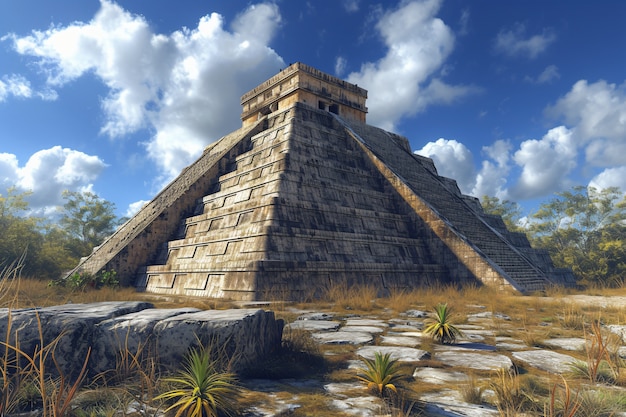The image features an ancient Mayan pyramid constructed from dark grayish stone, rising in tiered levels with a smaller square structure at the summit. The imposing pyramid, seen from an angle that reveals two sides, has central stairs ascending each tier. The scene is set outdoors on a bright day, under a blue sky dotted with patches of white and light gray clouds. The area surrounding the pyramid is dotted with lush tropical plants and trees, creating a verdant backdrop. The ground in the foreground is strewn with stones, laid out in a manner suggesting an old, purposefully placed pathway. Among these stones, a particularly large, partly flattened one stands out, possibly a man-made bench or an intentionally shaped rock. The pyramid and its surroundings appear weathered and worn, attesting to their ancient origins. The vivid greenery and the clear sky encapsulate the serene yet majestic essence of this historic site.